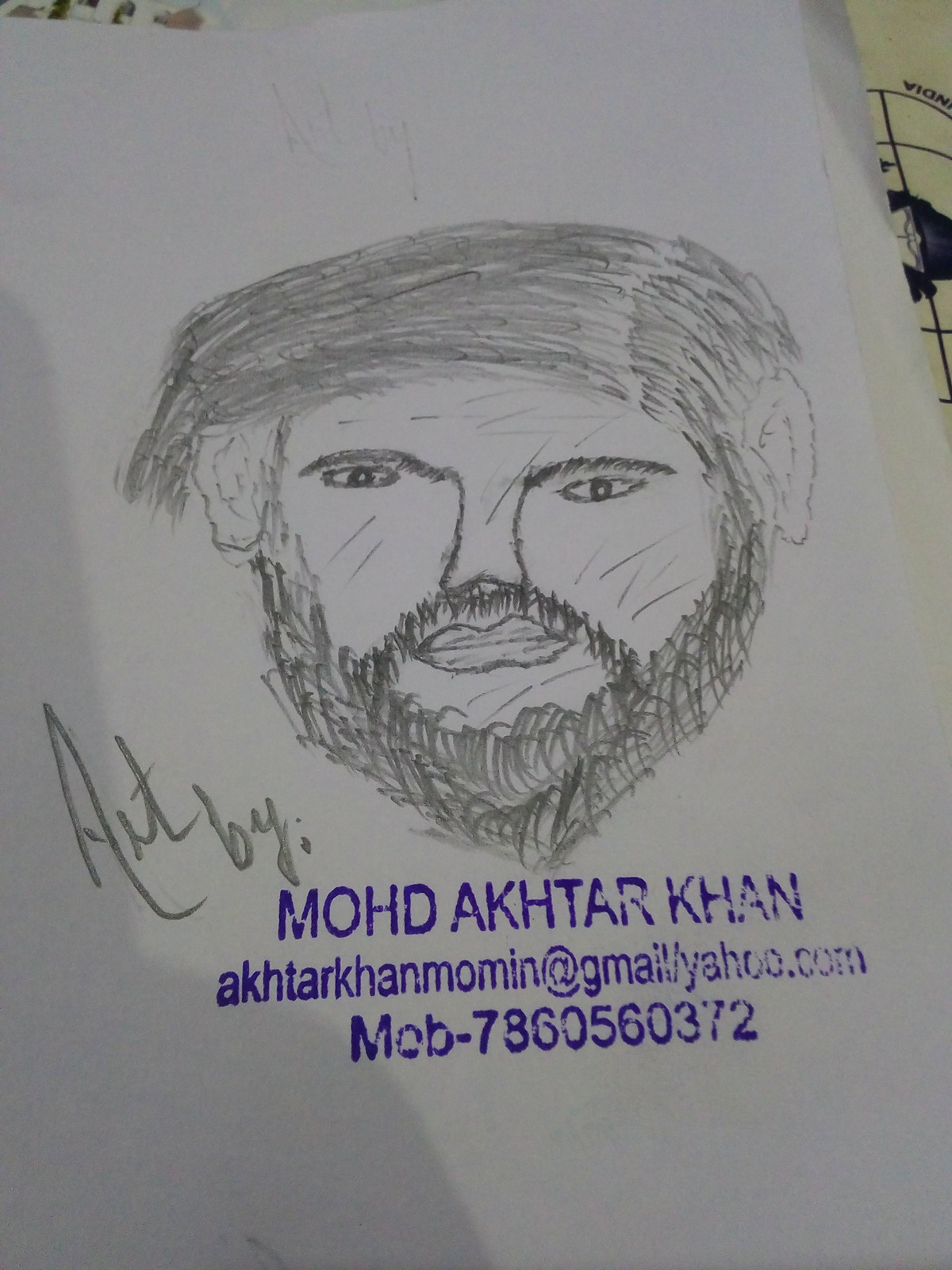The image showcases a detailed black and white drawing on white paper, centered around the face of a person. The artwork meticulously captures his facial features, including his ears, eyes, eyebrows, hair, nose, mouth, beard, and mustache. In the bottom left corner of the face, there is a black initial. Beneath the face, there is text in purple ink that reads "MOHDAKHTARKHAN" and further below, "AKHTARKHAN."